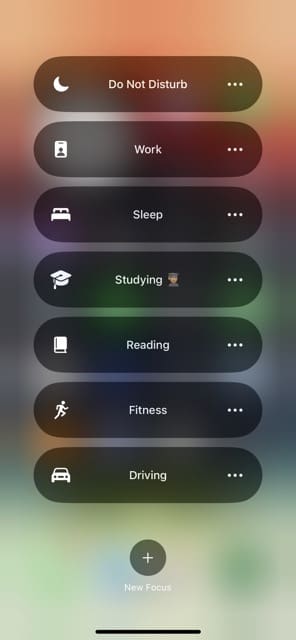The background of the image transitions through a spectrum of colors from top to bottom: starting with an orange-red at the top, blending into purple, then green, followed by a hint of orange, returning to green, and finally ending with touches of yellow and blue at the bottom. Against this colorful backdrop, several black ovals are vertically stacked. 

Inside each oval, there are different icons paired with text labels and ellipses:

1. The topmost oval features a crescent moon icon with the text "Do not disturb..."
2. Below it, a white badge icon labeled "Work..."
3. Next, a white bed icon denoted as "Sleep..."
4. Underneath that, a white graduation cap icon alongside the word "Studying..." and an emoji of a person with tan skin, wearing a black cap and gown.
5. Following that, a flat book icon with the text "Reading..."
6. Next is an animated figure icon, characterized by a simple circle for a head and an active pose with one arm and one leg raised, labeled "Fitness..."
7. Lastly, a white car icon with the label "Driving..." 

At the very bottom, the text "New Focus" is prominently displayed in white.